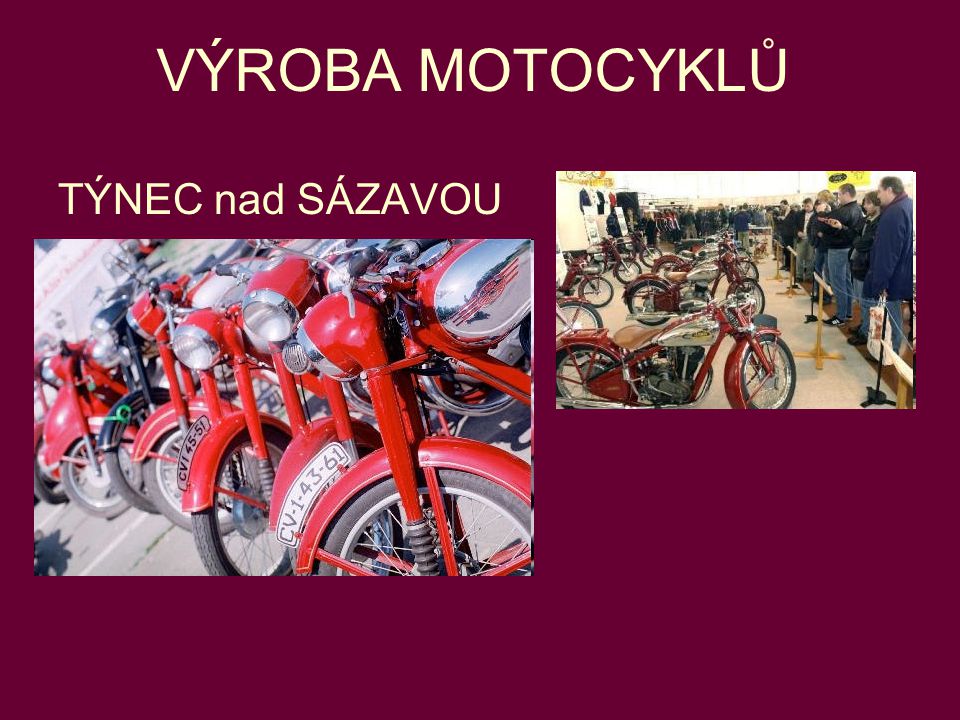The poster features a solid rectangular background in a shade of purple or maroon. At the top, centered, there's white text in all caps displaying "V-Y-R-O-B-A M-O-T-O-C-Y-K-L-U," with the "Y" and "U" accented, indicating a language other than English. Below this, aligned to the left, there is more white text reading "T-Y-N-E-C N-A-D S-A-Z-A-V-O-U."

In the center of the poster, two rectangular images are arranged. The larger image, positioned on the left, shows a close-up view of several red motorcycles lined up, focusing on their front tires and headlights. These motorcycles have an antique appearance, with prominently placed silver detailing around the gas tanks and license plates such as "CV-14361." The smaller image on the right depicts an indoor scene where a group of people stands behind a rope barrier, admiring these lined-up red motorcycles, reinforcing the idea that this is an exhibit of antique bikes.